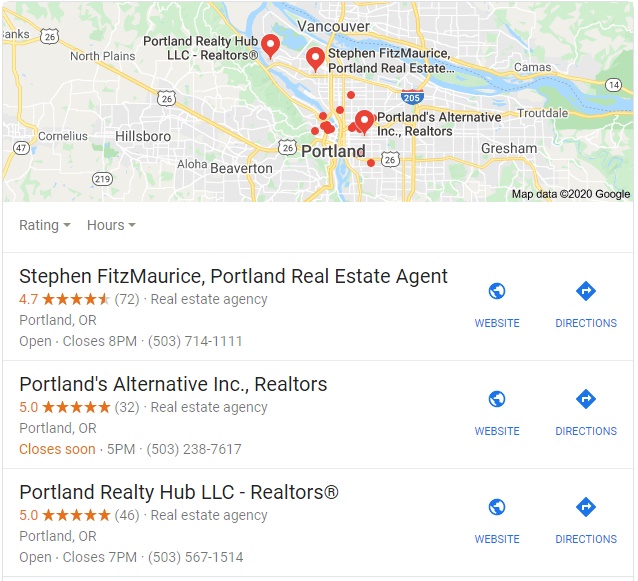This image appears to be a detailed screenshot from a real estate search platform focusing on realtors within the state of Oregon, particularly around the Portland area. At the top third of the image is a colorful map featuring several red dots, which likely denote realtor office locations. Three prominent, larger dots on the map correspond to detailed listings of three specific realty companies below. The map, extending from a portion of Vancouver down to Portland, highlights main thoroughfares such as Highway 14 running off to the left and Highway 26 extending past Hillsboro to the left side of the image.

The detailed listings for the three realty companies include:
1. **Stephan, Fitz, Muris, Portland Real Estate Agent**:
   - Contact Information
   - Website link
   - Directions

2. **Portland's Alternative Incorporated Realtors**:
   - Address
   - Phone number
   - Website link
   - Directions

3. **Portland Realty Hub LLC Realtors**:
   - Contact Information
   - Website link
   - Directions